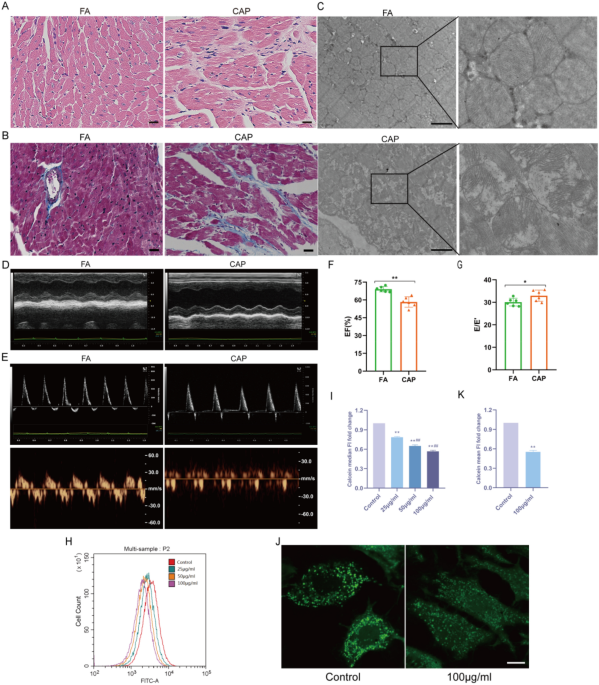The image features a grid of various small square and rectangular visual representations, organized systematically from top to bottom and left to right. In the upper left corner, a figure labeled "A" comprises four squares, with two shaded mostly in purple accompanied by gray lines, and two in light gray. Directly below, figure "B" contains two squares in darker purple with gray, and another two in gray. The next row down, labeled "D," has two black and white images that seem to be highly magnified, followed by two black rectangles with irregular peaks against a black background. The subsequent row marked "E" displays two rectangular images with peaks and valleys, reminiscent of signal waves, and two more rectangles below this row showing gold lines, potentially spectral lines. To the right of this section, four bars charts are present though the axes' details are illegible. In the lower left corner, a line graph ascends to a peak, while in the lower right, two additional black squares with highlighted green areas are seen. Labels "H" and "J" are attached to the squares in the bottom row, which include green patterns on black backgrounds, and one is noted as marked "control," suggesting it may be an experimental setup.